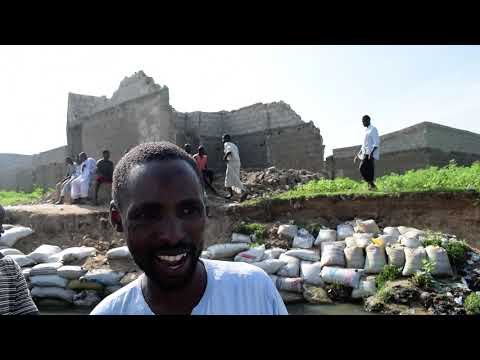The image shows a dark-skinned black man in the foreground, captured from the armpits up. He is smiling broadly, possibly laughing or talking, and looking slightly off to his left. He has very short hair and may have a mustache or a beard, though the details are obscured due to the sunlight coming from behind him to the right. He is wearing a white t-shirt. Behind him, there is a wall lined with sandbags, suggesting a protective measure against potential flooding. Above the sandbags, an embankment leads to a grassy area. In the background, partially destroyed or decaying buildings are visible, with just the walls remaining amid rubble. Around a dozen other black individuals are either sitting or standing near the building or in the grassy field to its left and right, creating a scene of communal interaction or shared activity amidst the ruins.